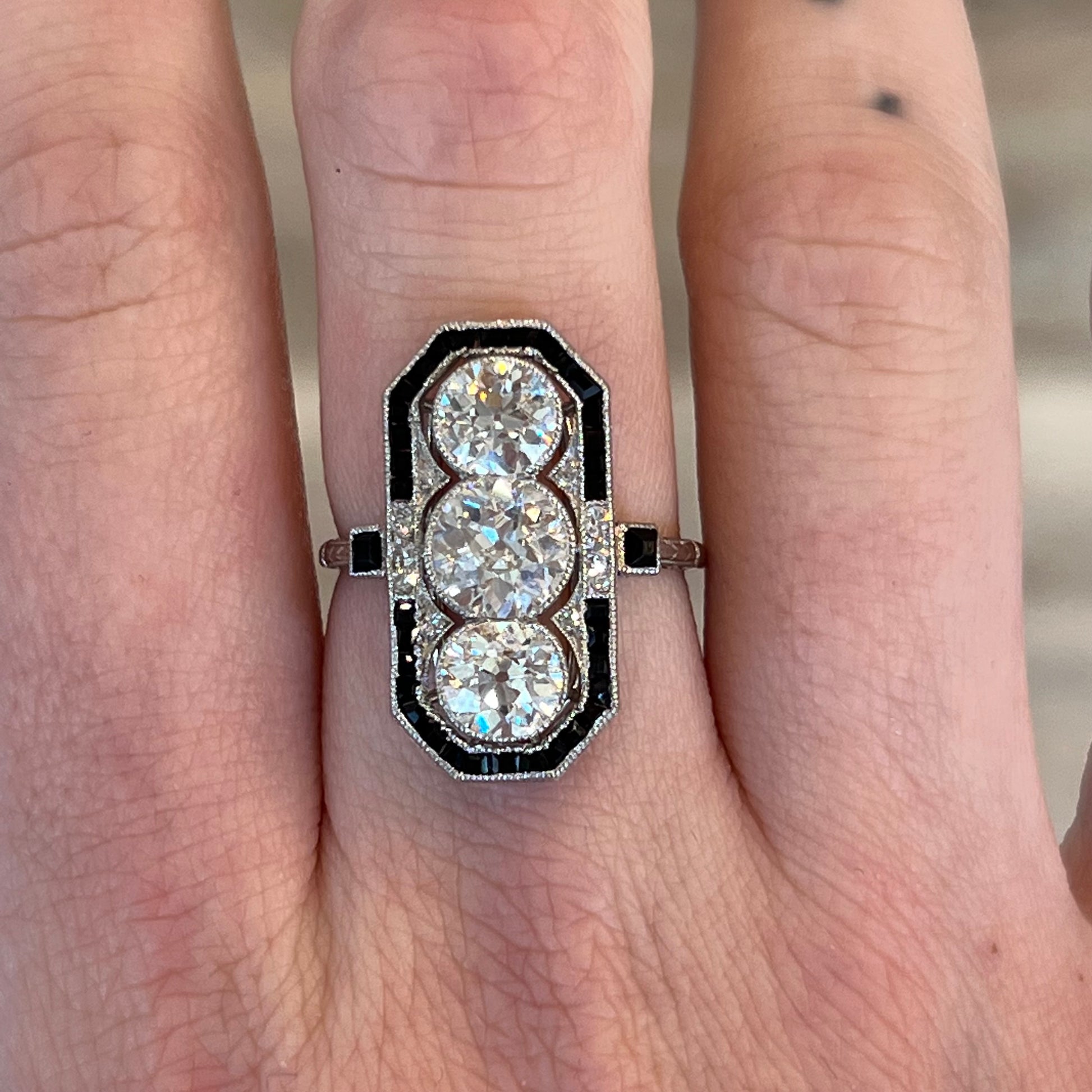This close-up photograph captures an absolutely stunning ring on the middle finger of a white person's hand. The hand, adorned with a tattoo on one knuckle and some hand wrinkles and ink smudges, serves as the perfect backdrop for the intricate piece of jewelry. The ring itself is an art deco style masterpiece, featuring three large, brilliantly shimmering circle diamonds arranged vertically down the center. These diamonds are engulfed by an almost coffin-shaped border of dark gemstones, likely black onyx or deep sapphires, which extend along the vertical axis from the knuckle to the base of the finger. The ring is further accentuated by two smaller, square gemstones on each side. The light reflecting off the various stones creates a mesmerizing display of pinks, blues, and greens, highlighting the ring's exquisite detail and craftsmanship. The blurred background keeps the focus solely on the dazzling, glimmering gemstones of the ring.